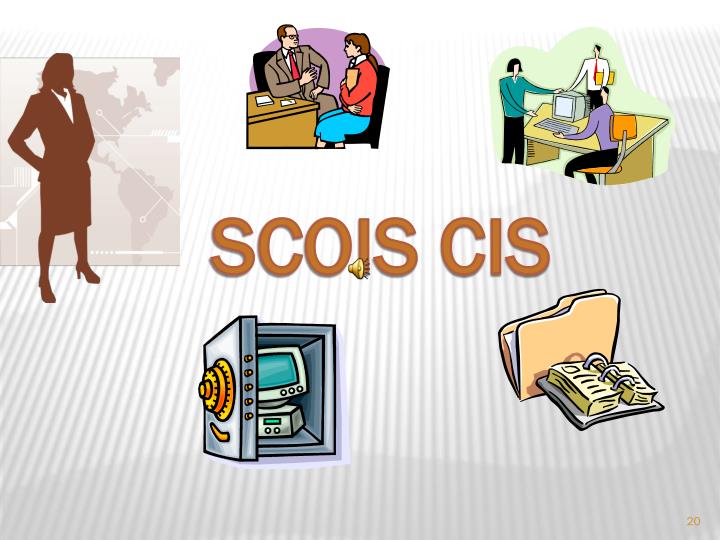The image is a digitally created clip art illustration set against a tan and white striped background. In the center, there is text in brown and gold lettering that reads "SCOIS CIS," with the first "I" featuring a small, sideways bell icon. The illustration is composed of several cartoon-like elements: 

- **Top Left:** A brown silhouette of a woman in a business suit dress stands in front of a dimly lit map of North and South America.
- **Top Center:** A man in a business suit is seated at a desk, conversing with a woman who appears to be a secretary, holding a folder.
- **Top Right:** Three individuals are clustered around a computer desk, one is seated in an orange chair, the others are standing, with one holding papers.
- **Bottom Left:** An open vault containing a computer.
- **Bottom Right:** A daily planner next to a file folder.

The overall color palette includes shades of brown, gray, white, orange, yellow, purple, red, turquoise, and light blue. The objects are scattered around the central text, creating an organized collage effect, suggesting the image might be part of a presentation slide.